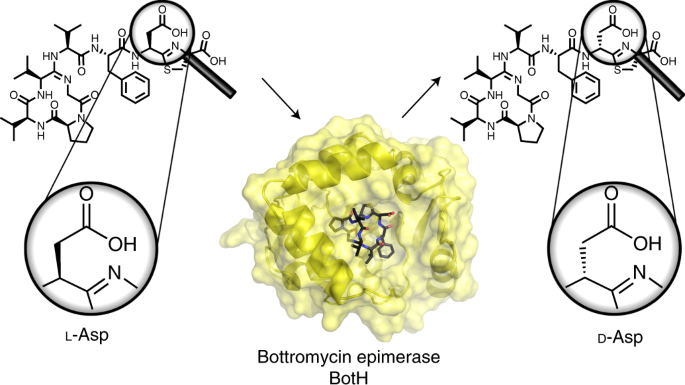The image is a detailed textbook diagram depicting the chemical structure and relationship between different parts of botromycin epimerase (BOT H). At the center of the image is a yellow, cream cheese-like mass with small blue, red, and black elements, labeled "BOT H." Above this mass is a magnified black and white random shape, illustrating a portion of the molecule.

On the left side of the diagram, labeled "L-Asp," there is a close-up of the molecule's bond structure featuring oxygen (O), hydrogen (H), and nitrogen (N) atoms. This section is connected to the central BOT H mass with an arrow pointing toward it, indicating a reaction or interaction.

Similarly, the right side of the diagram showcases another close-up, labeled "D-Asp," depicting similar molecular components (O, H, and N) but illustrating a different structural arrangement. This section has an arrow pointing from the central BOT H mass to the right, indicating a chemical transformation or pathway.

Additionally, the depiction includes two main circles, one at the top and the other at the bottom right side, connected by lines, resembling a pulley system. These circles and their connections likely represent the cyclic nature of the molecular interactions or processes. The entire diagram thus effectively demonstrates the distinction and relationship between L-Asp and D-Asp forms of the molecule and their connection to botromycin epimerase.